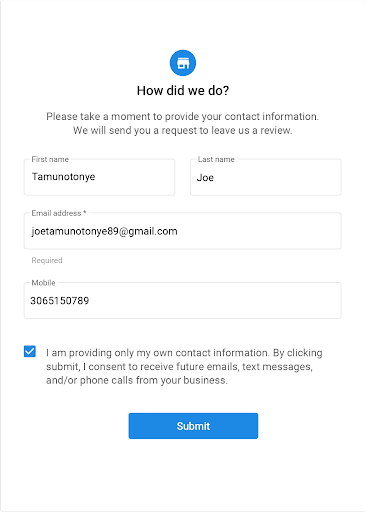The image features a form with a clean, white background. Centrally positioned at the top is a blue circle containing an indistinguishable white icon. Directly beneath the icon, the text reads "How did we do?" and is followed by a request: "Please take a moment to provide your contact information. We will send you a request to leave us a review.”

Below this prompt, there is a series of text boxes for user input:

1. **First Name**: The placeholder text within the box is "T-A-M-U-N-O-T-O-N-Y-E."
2. **Last Name**: To the right of the first name box, with the placeholder text "Joe."
3. **Email Address**: Underneath the first name field, it displays an example email address, "JoeT-A-M-U-N-O-T-O-N-Y-E89@gmail.com," with a note indicating that this field is required.
4. **Mobile**: Directly below the email address field, the text box contains an example number, "306-515-0789."

The form is designed to collect feedback and contact information required to request a review from users.